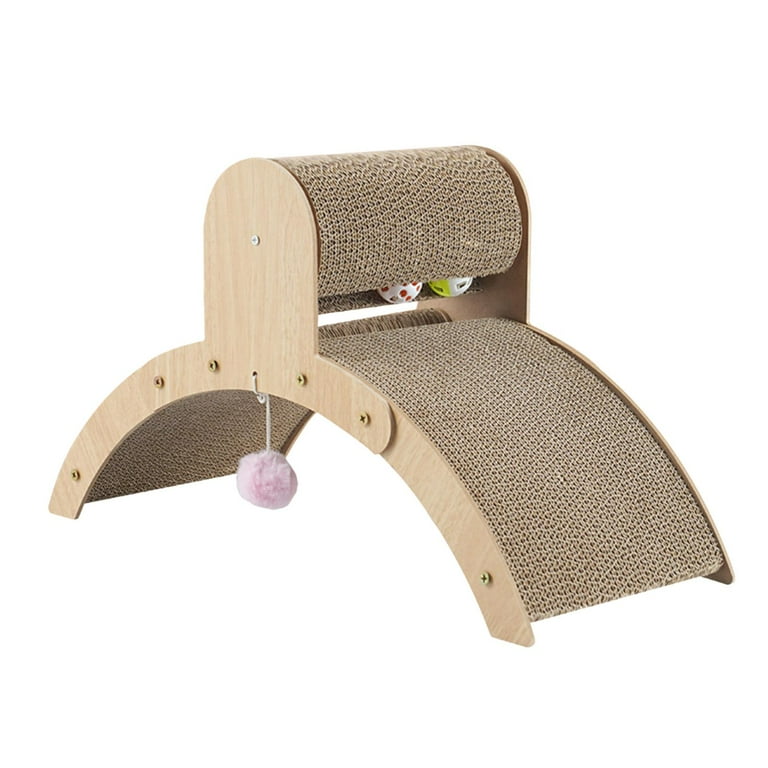The image depicts a unique and multifaceted cat toy and scratcher, designed with both play and practicality in mind. The central feature is an arching ramp, reminiscent of a rainbow, covered in scratch-friendly material, specifically tough corrugated cardboard or a scratchy carpet texture. This arch structure is bolstered on either side by smooth wooden edges, securely fastened with visible screws. The top of the arch boasts a cylindrical roller, similar to a car wash roller, inside of which two jingle balls—colors varying between white with green or orange, red, and yellow—are positioned to engage the cats. Suspended from the underside of the arch is a small, fuzzy, or foam ball, in a soft pink or lilac hue, adding another layer of interactive fun. This product, set against a clean white background, showcases a well-rounded play area encouraging cats to scratch, play with the balls, and swat at the hanging toy, making it a versatile addition to any cat's playtime provisions.